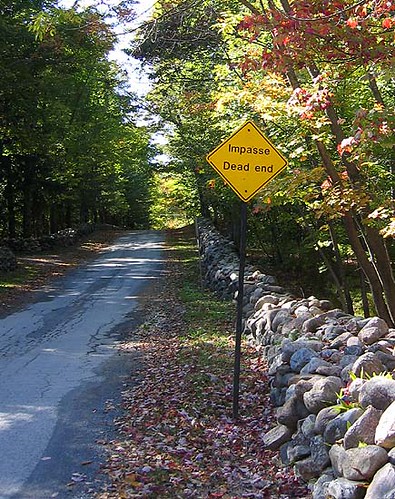The image depicts a rural, single-lane road surrounded by tall trees on both sides, with many leaves scattered on the ground, indicating the onset of fall. The road appears to be paved but shows signs of neglect, with numerous cracks and uneven edges. A prominent feature on the right side of the road is a yellow diamond-shaped caution sign mounted on a black metal pole, reading "IMPASS DEAD END," warning drivers that the road leads to a dead end. Adjacent to the sign is a dry-stacked rock wall, made up of large stones piled about 20 high, stretching along the road as far as the eye can see. The sky is visible through gaps in the tree canopy, hinting at a clear, blue day. Despite the maintained patches, the road's aged appearance suggests it has been in place for quite some time.